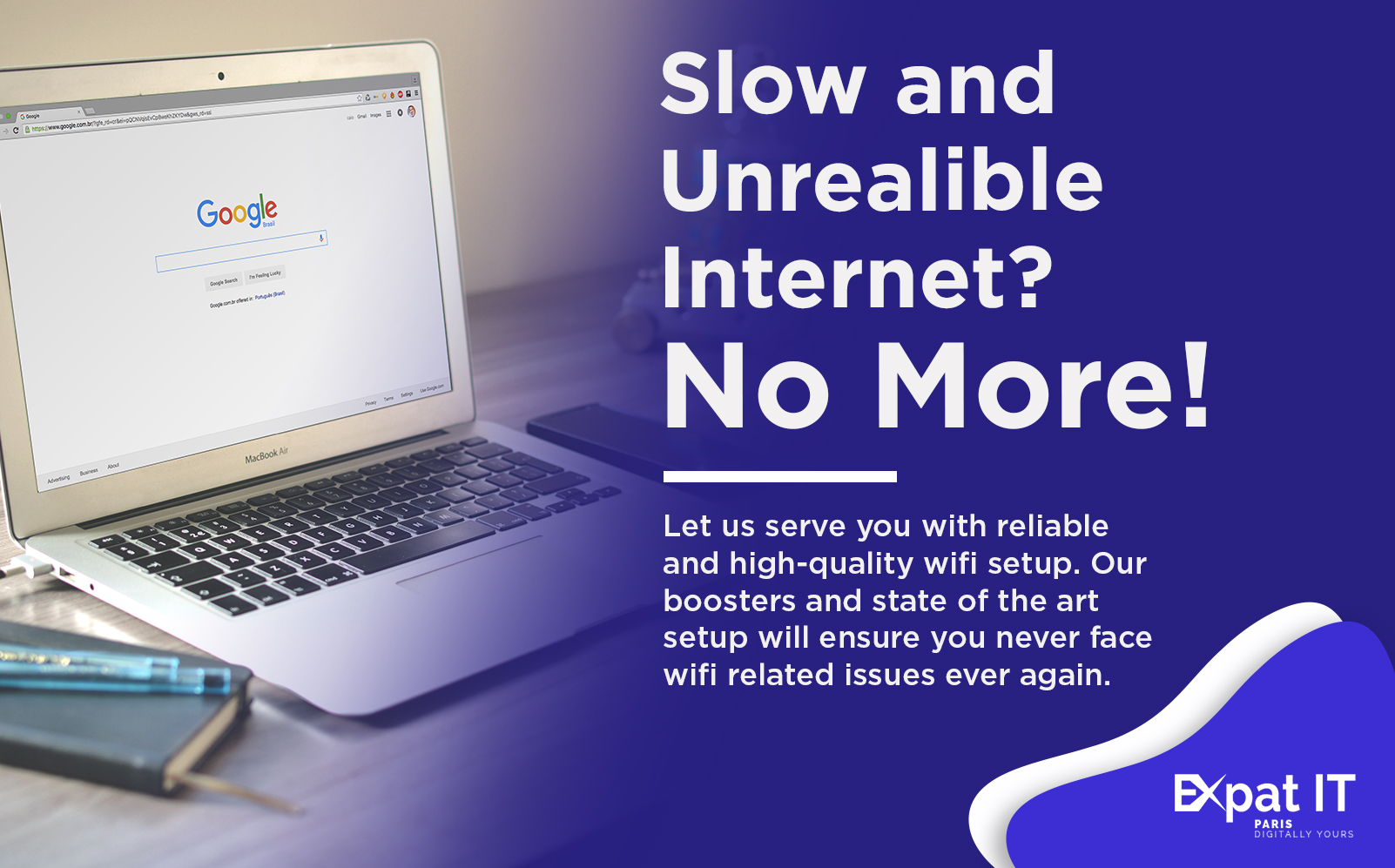This horizontally aligned rectangular image features a silver MacBook on the left side, opened to display the Google homepage with its distinctive multicolored logo and search bar on a white screen. To the left of the MacBook, there is a small closed notebook with a pen resting on top, set against a grayish background. The image transitions from a purplish color that fades into yellow on the left, to a dark blue background on the right. The right-hand side of the image prominently displays white, left-aligned text reading, "Slow and unreliable internet? No more!" The phrase "No more" is emphasized with slightly larger letters. Below a small horizontal white line, additional text reads, "Let us serve you with reliable and high-quality Wi-Fi setup. Our boosters and state-of-the-art setup will ensure you never face Wi-Fi related issues ever again." In the bottom right-hand corner, there is a curved blue and white graphic with the text "Expat IT" and "Paris," indicating an advertisement for internet service.